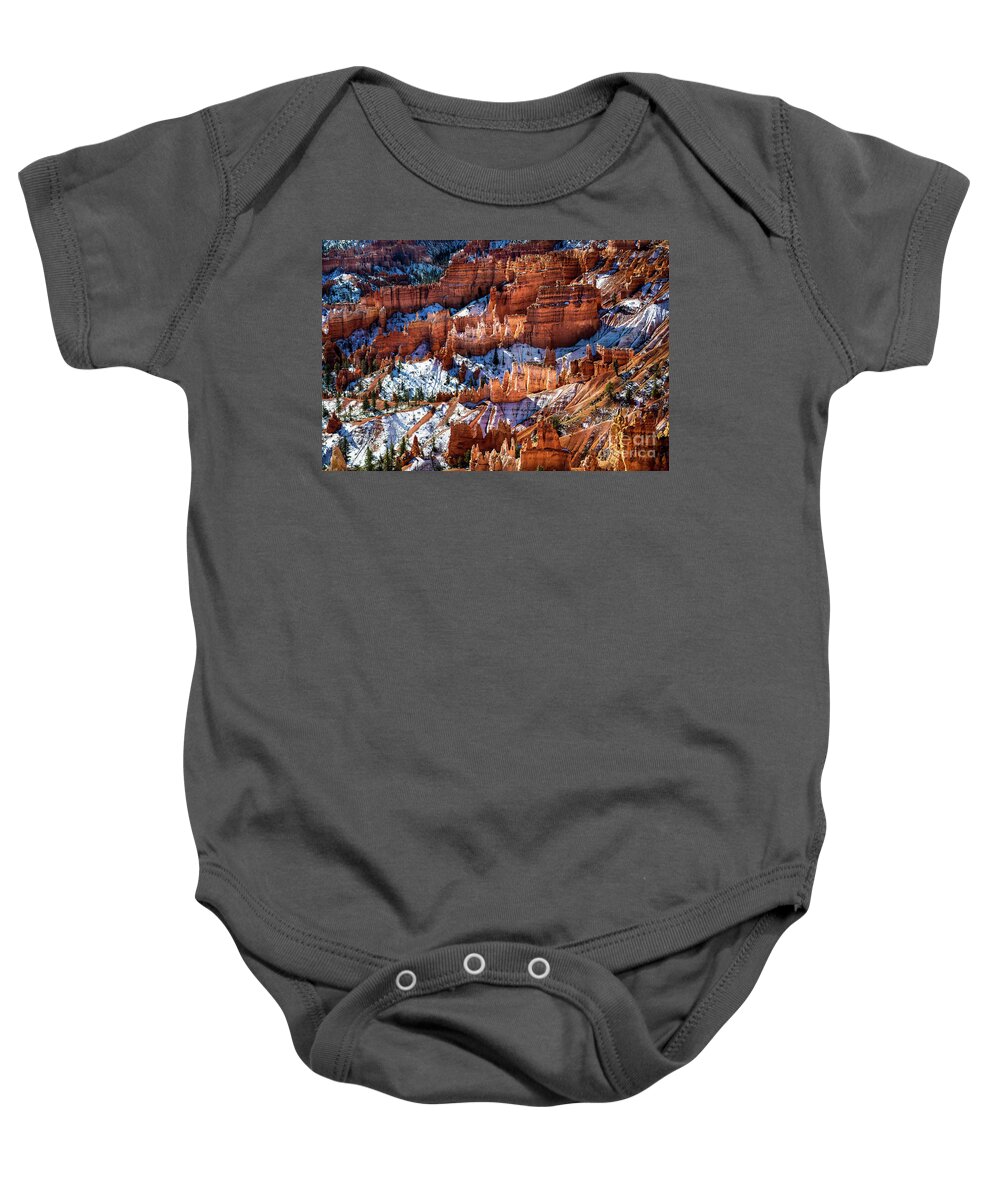This photograph features a dark gray baby onesie, laid out with its short sleeves spread to the sides. Prominent at the bottom are three silver snap buttons used to secure the onesie around the legs. The onesie, designed for a larger baby rather than an infant, sports a rounded neck with subtle gusseted shoulder slits for added comfort and mobility. At the center of the chest is a rectangular image depicting an abstract, snowy canyon landscape. The scene within the print includes layered canyon walls in various shades of brown and red, dusted with white snow and accented with patches of green trees. Small text, likely a watermark reading "Find Art America," is faintly visible in the bottom right corner of the image. The overall wrinkle pattern near the neckline and around the stomach to crotch area adds a touch of realism to this visually detailed garment.